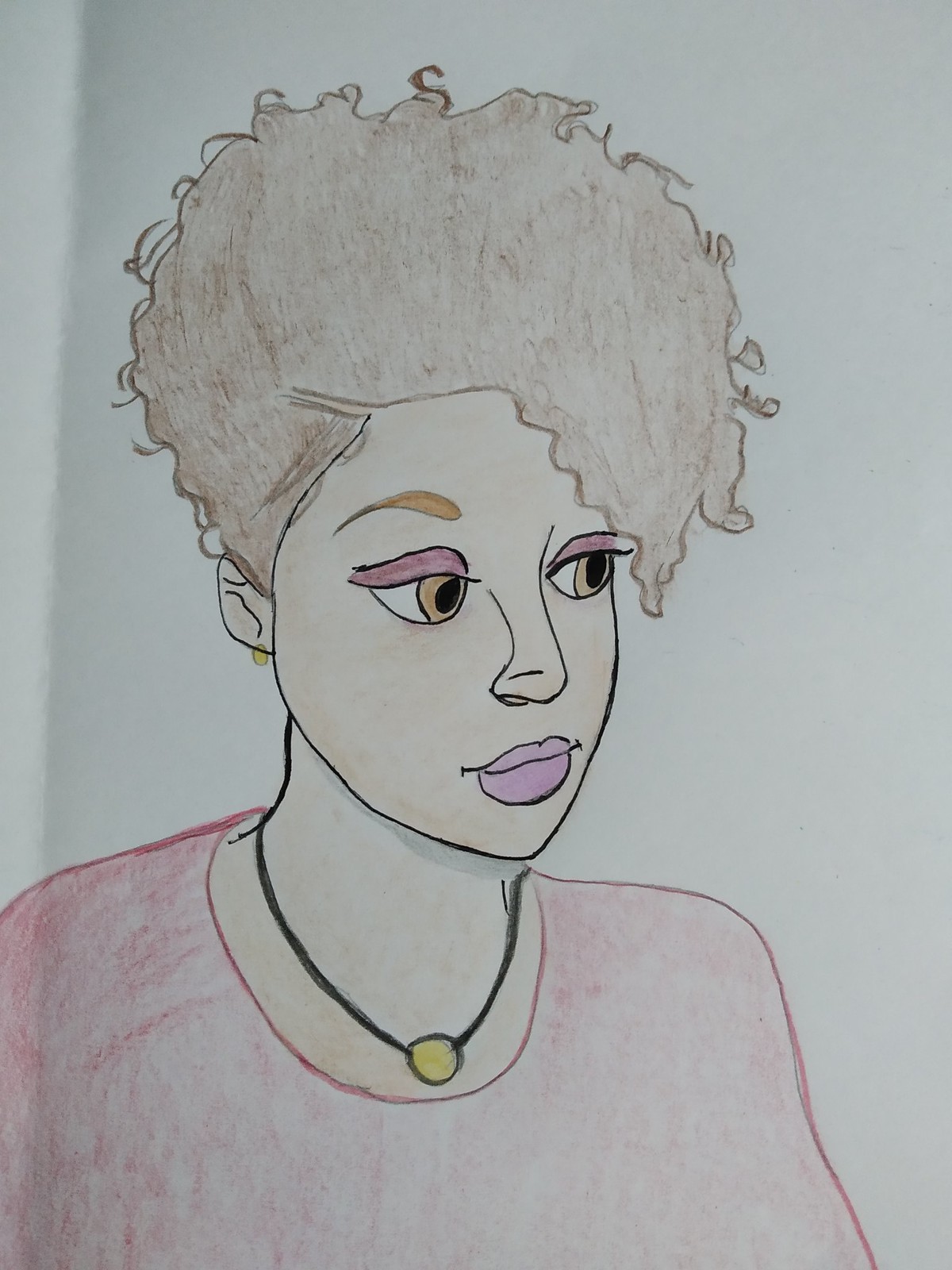This image depicts an artistic drawing of a woman, portrayed from the shoulders up against a stark white background. She is adorned in a reddish-pink sweater, complementing her light skin tone that shows hints of melanin, suggesting a mixed ethnicity, likely part African American and part European. Around her neck hangs a small choker necklace on a black string, featuring a yellow circular pendant as its centerpiece.

Her brown hair is styled in a short, curly fashion, cascading slightly over her forehead while gathered in an intricate up-do that accentuates her unique look. Her eyes, large and light brown, are a focal point, set under expressive, lightly colored eyebrows with an orange hue. She gazes thoughtfully to the right, enhancing the contemplative and happy ambiance of the portrait.

The woman’s makeup features pink eyeliner and eye shadow, complementing her full, pink lips. The detailed rendering, which blends sketching with subtle coloration, captures not only her appearance but an essence of depth and personality.